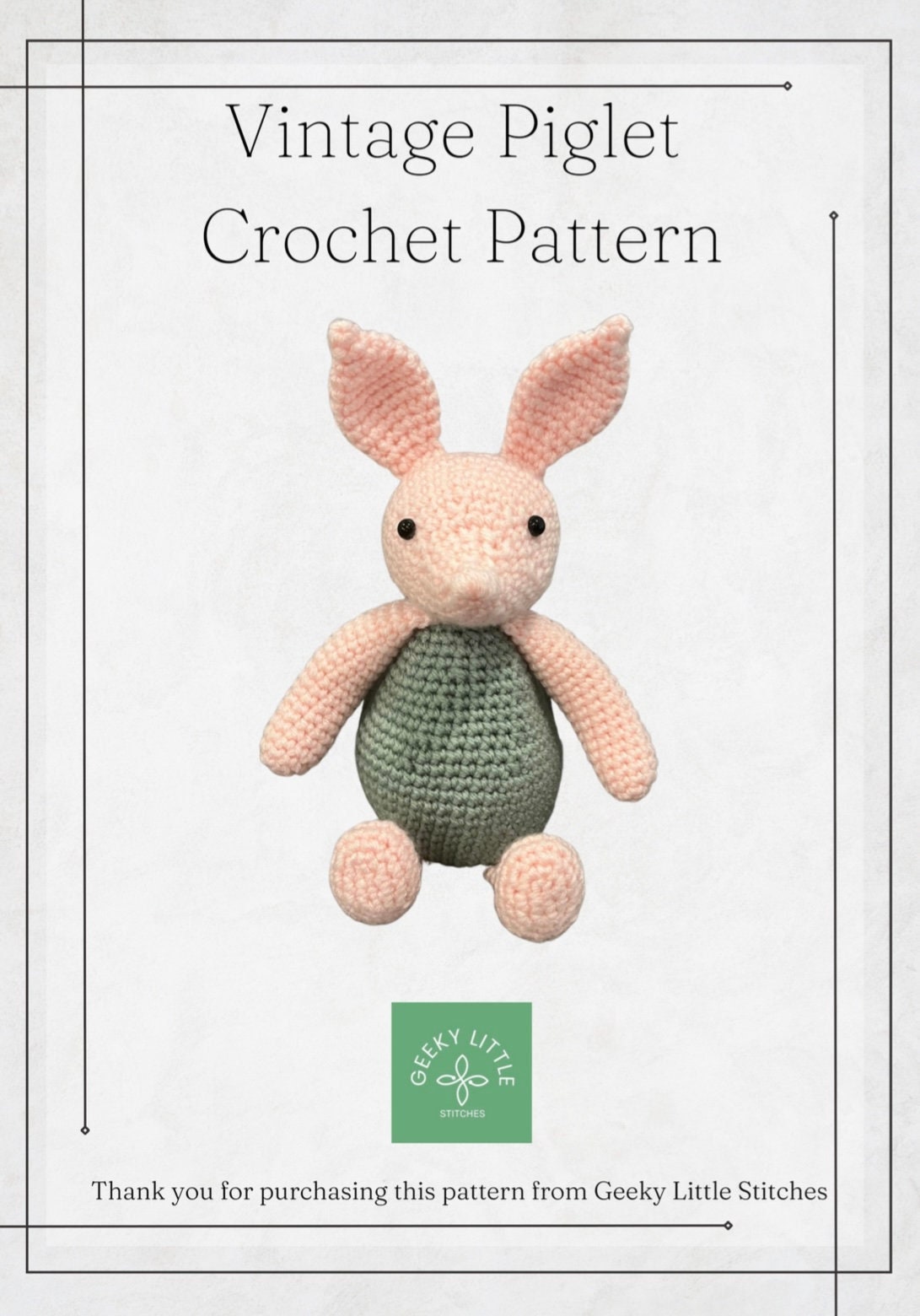This image showcases a "Vintage Piglet Crochet Pattern" against a slightly dull white background. Central to the image is a crocheted piglet with a pink head, ears, arms, and legs, distinguished by small black dot eyes. The piglet's torso stands out in a light green color. Surrounding this artwork are broken, dotted black lines forming a rectangular border. At the bottom of the image, there's a logo within a light green square featuring a stylized flower and the text "Geeky Little Stories" written in white. Beneath this, in black text, the image reads, "Thank you for purchasing this pattern from Geeky Little Stitches."